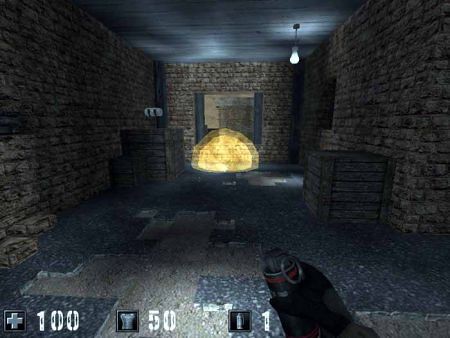In this video game screenshot, a character stands at the end of a narrow, dead-end alley flanked by brick walls. On the right side of the alley sits an old wooden crate, while two more wooden crates are positioned on the left. At the end of the alley, a vibrant orange explosion unfolds, adding a sense of imminent danger. From the bottom right corner of the screen, a gloved hand extends into view; the glove is black with a gray top. The hand clutches a cylindrical object that resembles a hand grenade or gas canister, complete with a pull ring and a surface marred by large square indentations. In the bottom left corner of the screen, a HUD (Heads-Up Display) shows a plus sign next to the number 100, accompanied by a block with a shirt icon and the number 50, followed by another block displaying the number 1.